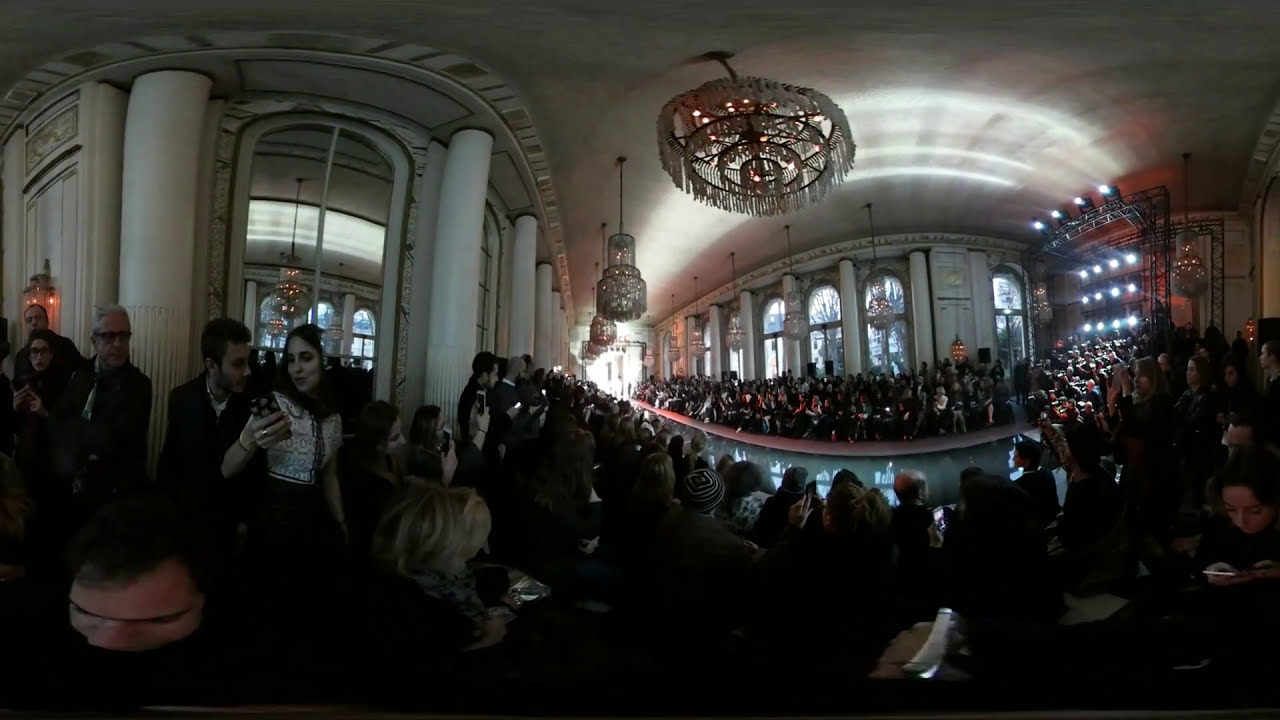This photograph depicts the interior of an elegant, expansive building, possibly a church or grand hall, hosting what appears to be a fashion show. The wide-angle, possibly manipulated shot captures a turquoise blue runway cutting through rows of people, indicating the area where models would typically walk. The room is crowded with individuals, many dressed in suits and some engrossed in their phones. Ornate chandeliers hang from the high ceiling, enhanced by beams and poles adorned with additional chandeliers, casting a sophisticated glow. The background features unique oval windows, adding natural light to the otherwise dimly lit space. A couple on the far left catches the eye; the woman looks at her phone while the man gazes at her. The overall ambiance is one of anticipation, as the seated and standing attendees await the start of the event.